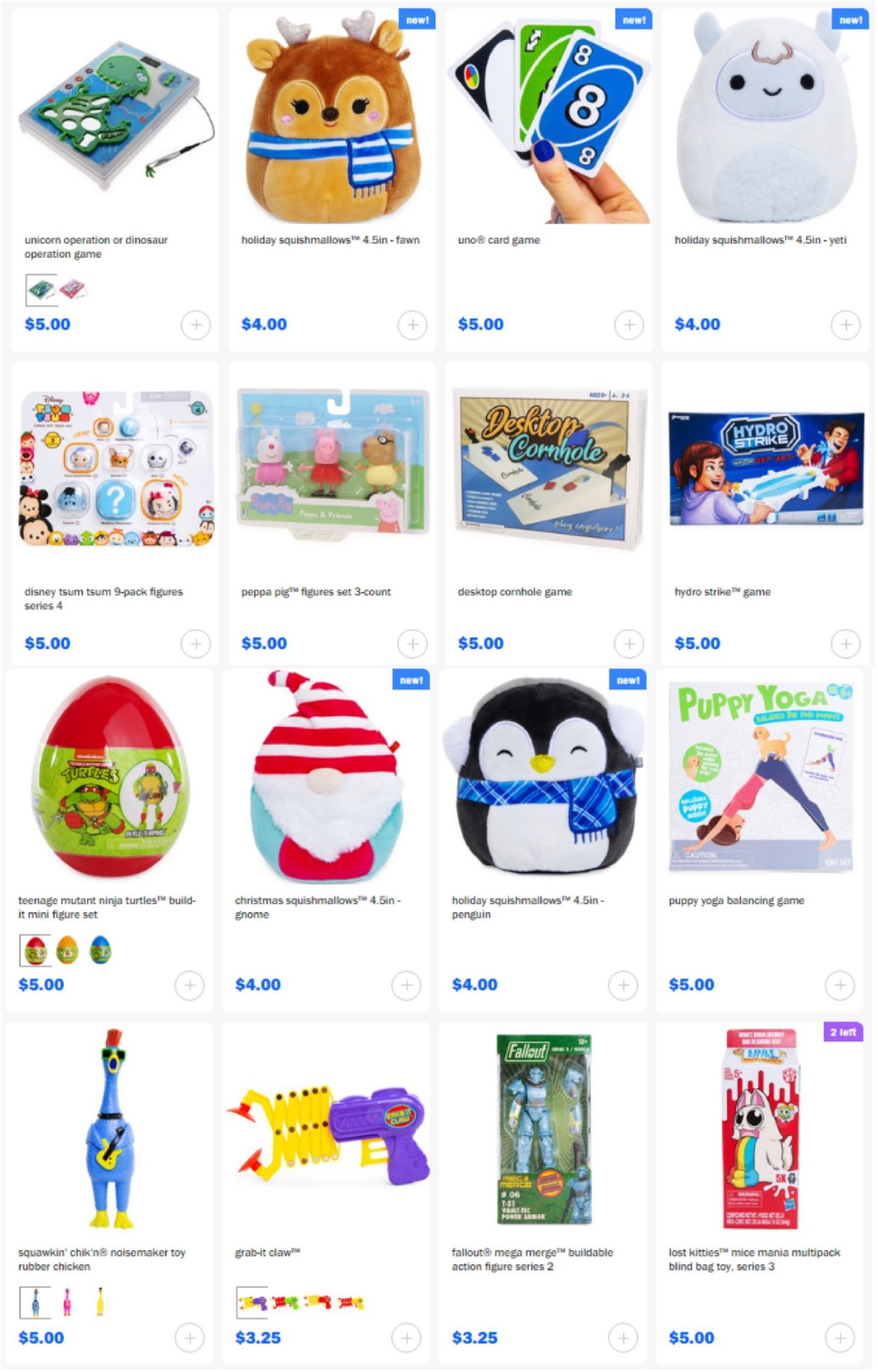This is an organized image showcasing a variety of toys and games displayed on a retail website, arranged in a portrait-oriented, four-column grid. Each column contains three items housed in white, portrait-oriented rectangular boxes with subtle gray borders. The first column features a "Unicorn Operation on Dinosaur" board game for $5, a Squishmallow plush toy for $4, and an Uno Card Game for $5. In the second column, there are Holiday Squishmallows for $4, a Disney 9-Pack Figures set for $5, and Peppa Pig Figures 3-Set Count for $5. The third column displays a Desktop Cornhole Game for $5, a Hydra Strike game for $5, and the Teenage Mutant Ninja Turtles Building Minifigures Set for $5. The fourth column includes Christmas Squishmallows for $4, a book called "Puppy Yoga Balancing Game" for $5, and a Squawkin' Chicken Noisemaker Toy Rubber Chicken for $5. Items continue with a Grab It Claw game for $3.25, a Fallout Mega Game Bundle Action Figure Series for $3.25, and a Lost Kitties set for $5. Each product image is clear, and the prices hint at a discount retail setting, suggesting that this may be an online discount store, offering competitive prices significantly lower than typical retail prices.